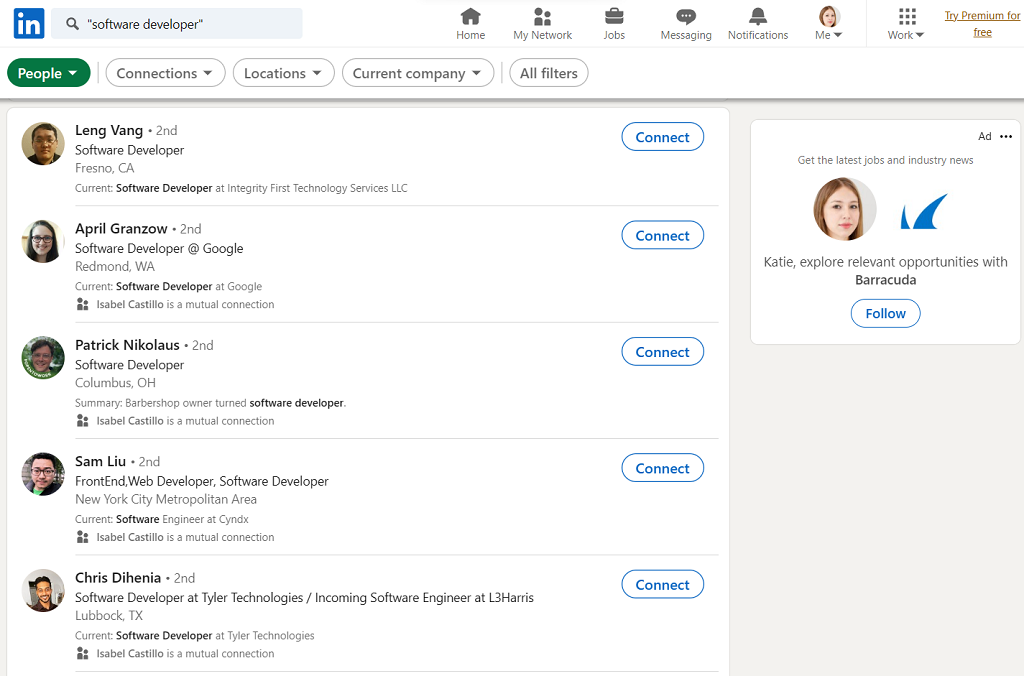Here is the cleaned-up and detailed caption:

---

This LinkedIn screenshot features a clean, white background with the LinkedIn logo—a blue square with the lowercase letters "in" in white—situated in the upper left corner. Prominently positioned at the top of the screen is a light gray search box containing the search term "software developer" enclosed in quotation marks.

On the right side of the navigation bar, various menu items are listed: Home, My Network, Jobs, Messaging, Notifications, and Me, which is accompanied by the user's profile photo. The photo depicts a young Asian woman in her 20s with reddish-brown hair. Adjacent to this is the "Work" section.

Beneath the menu, there's a larger version of the same profile photo next to a call-to-action that reads, "Get the Latest Jobs and Industry News." Beneath this header, there's personalized text: "Katie, Explore Relevant Opportunities with Barracuda," followed by a blue "Follow" button within a rounded rectangle.

The left side of the screen displays search results for "software developer," listing five individuals with their profile photos and names. Each profile entry includes a blue "Connect" button enclosed in a blue rectangle with rounded corners. The five profiles shown are:

1. Ling Vong
2. April Guangzhou
3. Patrick Nicholas
4. Sam Liu
5. Christopher Dihenia

---

This structured and detailed description captures all the elements present in the original screenshot.